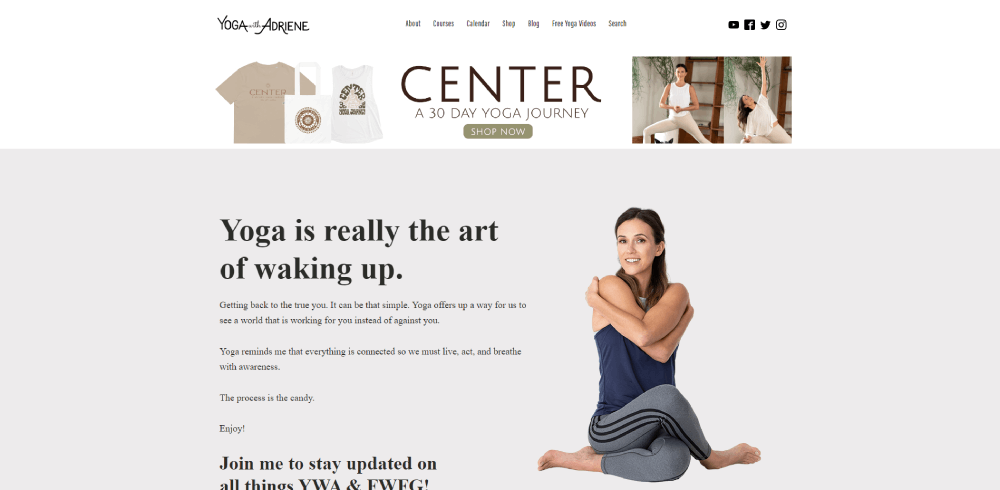In the image, the top left corner features "Yoga with Adriene," a website offering various resources such as courses, a calendar, a shop, a blog, free yoga videos, and a search function. Toward the top right, there are icons linking to YouTube, Facebook, Twitter, and Instagram. Centrally located is an invitation to embark on a 30-day yoga journey, accompanied by a "Shop Now" button. The image includes several visuals of people performing yoga poses, emphasizing the practice's elegance. A poignant caption reads: "Yoga is really the art of waking up. Getting back to the true you. It can be that simple. Yoga offers up a way for us to see a world that is working for you instead of against you. Yoga reminds me that everything is connected so we must live, act, and breathe with awareness. The process is the candy. Enjoy." The call to action encourages viewers to join Adriene to stay updated on all things related to Yoga with Adriene and the Find What Feels Good (FWFG) community. For more information, the website www.fweg.org is provided.